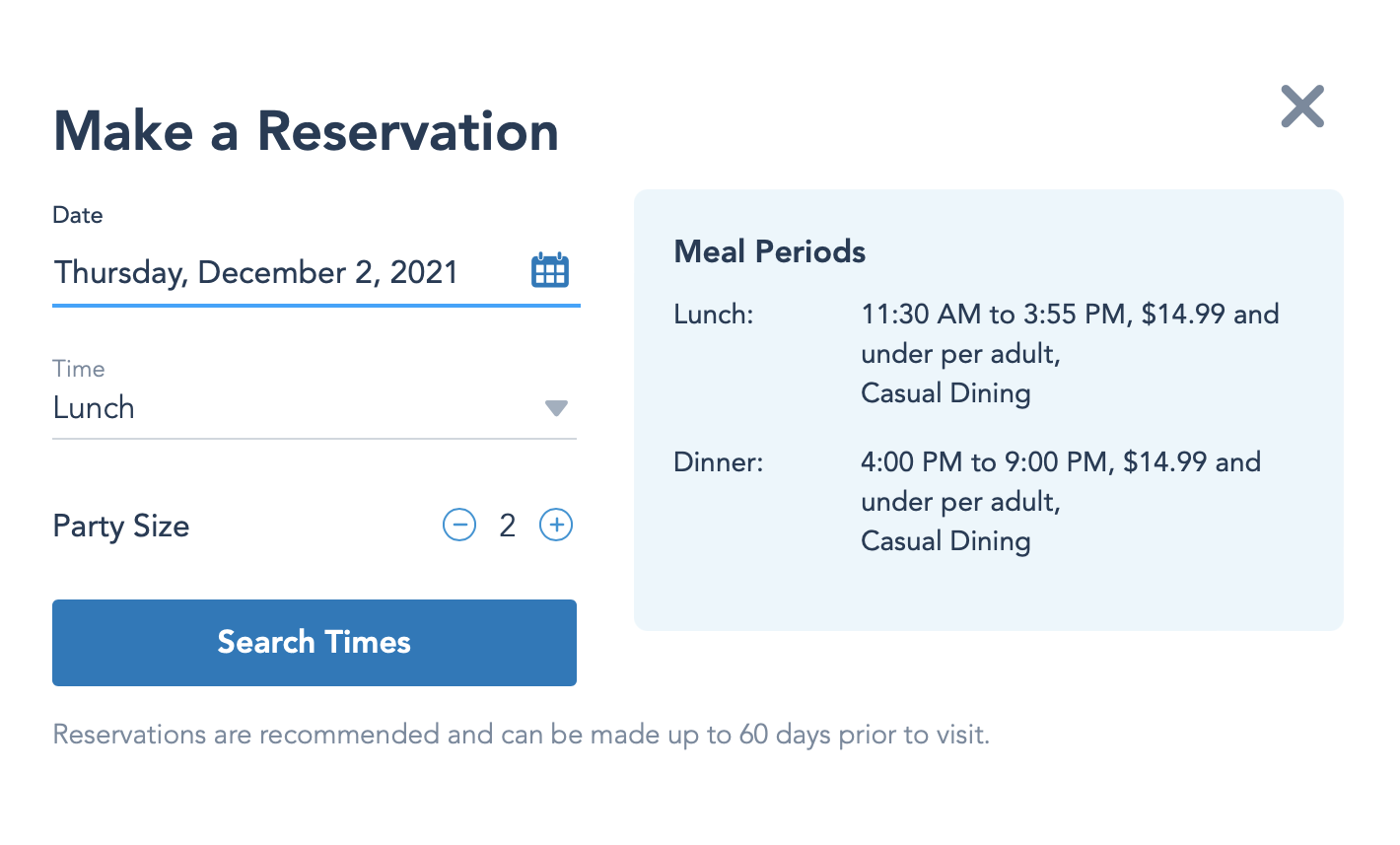This is a descriptive caption for the image of a website's reservation page:

---

The screenshot showcases a restaurant reservation webpage. On the top left corner, bold black text reads "Make a Reservation." Directly below, in smaller black text, is the label "Date." Beneath it, in gray letters, is the text "Thursday, December 2nd, 2021," accompanied by a blue calendar button to the right for date selection.

Further down, the section titled "Time" appears in light gray text, with a drop-down menu next to it displaying "Lunch" in darker gray text. Adjacent to it is a downward-facing gray arrow for altering the time slot.

Below the time options is a "Party Size" label in dark gray. To its right are toggle buttons for adjusting the number of guests: a blue circular button with a minus sign, indicating the ability to decrease the number of guests, followed by the number "2" in between, and a blue circular button with a plus sign to increase the number of guests.

At the bottom of the form is a "Search Times" button. Towards the right, there's a light blue rectangular section labeled "Meal Periods" in bold black text. Under this section, it specifies two dining slots:

- "Lunch: 11:00 AM - 3:55 PM, $14.99 and under per adult, Casual Dining"
- "Dinner: 4:00 PM - 9:00 PM, $14.99 and under per adult, Casual Dining"

This entire interface is designed to guide users through selecting their desired date, time, and party size for a restaurant reservation, along with providing information on meal periods and corresponding details.